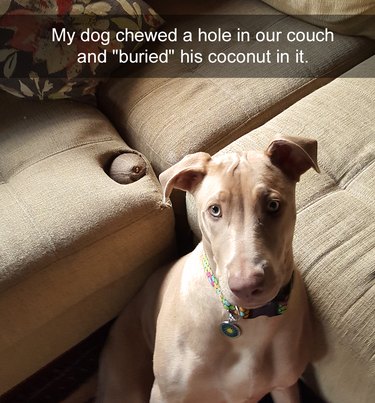In this vertically oriented rectangular image, a medium-sized dog sits in front of an L-shaped couch, looking directly at the camera with a guilty expression. The dog's light brown fur matches the light beige or tan sofa cushions behind him. He has large, floppy ears, a big pink nose, small sad eyes, and noticeable forehead wrinkles. The dog wears a green collar with a pendant featuring a yellow center.

The couch has three cushions, with the one on the left clearly showing a chewed hole, inside of which is a dog toy shaped like a coconut. This comical setting is enhanced by the text at the top of the image, in white Arial font against a semi-transparent dark bar, which reads: "My dog chewed a hole in our couch and 'buried' his coconut in it." The cushions and floral pillows form a V-shape behind the dog, emphasizing his central and remorseful placement in the scene.